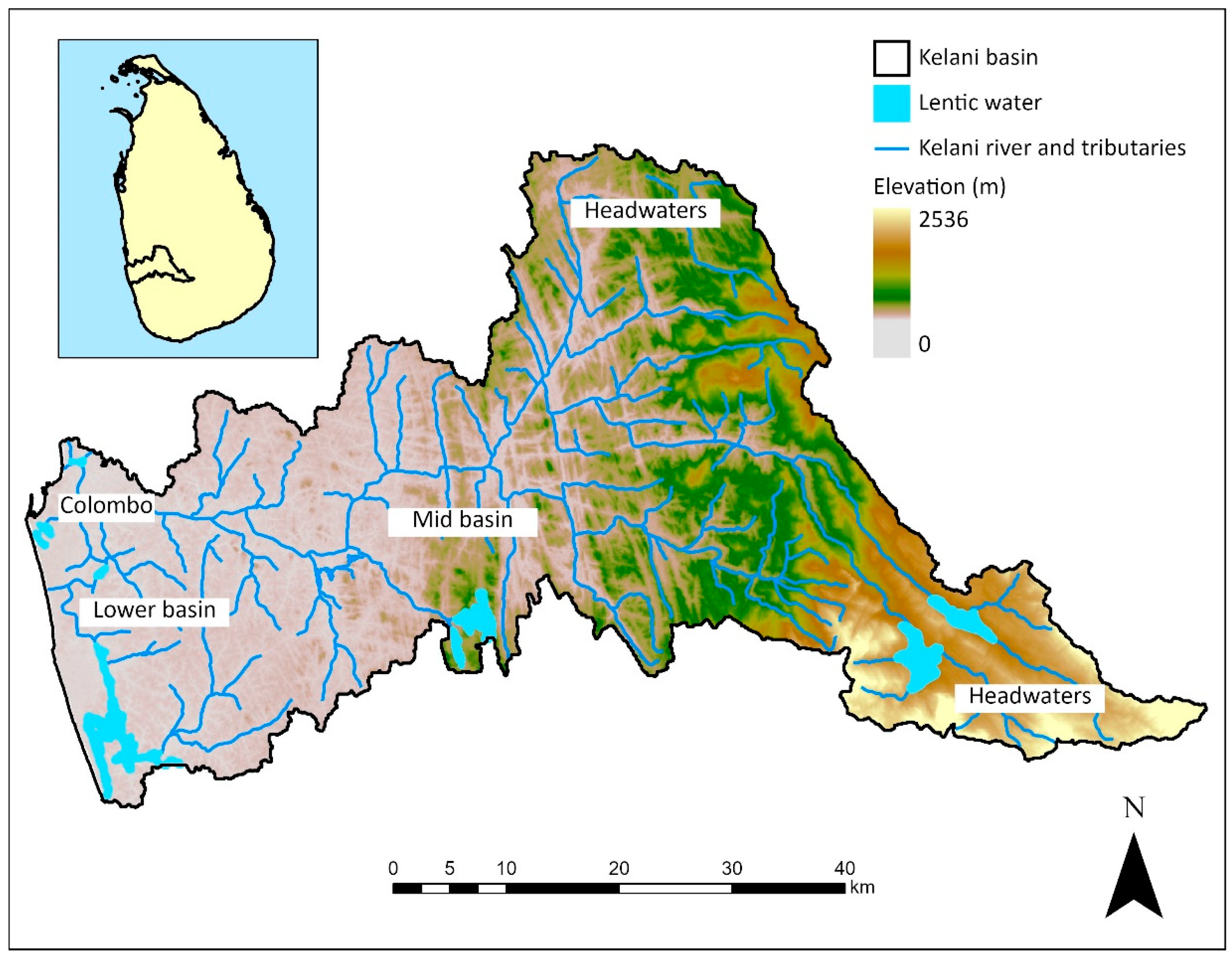The image depicts a detailed map with a white background and a landmass shaped oddly like a rotated boot. This map appears to focus on water flow, with several notable labels: “Headwaters” at both the top and bottom, “Colombo” and “Lower Basin” on the left, and “Mid-Basin” in the center. There are intricate river lines and an inset map at the top left indicating the larger geographical context.

The map includes a north arrow, a scale ranging from 0 to 40 kilometers, and an elevation scale indicating a range from zero to 2,536 meters. A legend at the top right specifies the Kalani Basin, Lentic Water, Kalani River, and its tributaries, along with color coding for elevation: pale pink transitioning through green, brown, and yellow hues. These colors and labels help illustrate the topography and water distribution across different regions.

In summary, this map visually represents the Kalani Basin's river systems and elevations, emphasizing various geographical features and water-related information through a combination of text labels, color scales, and detailed legends.